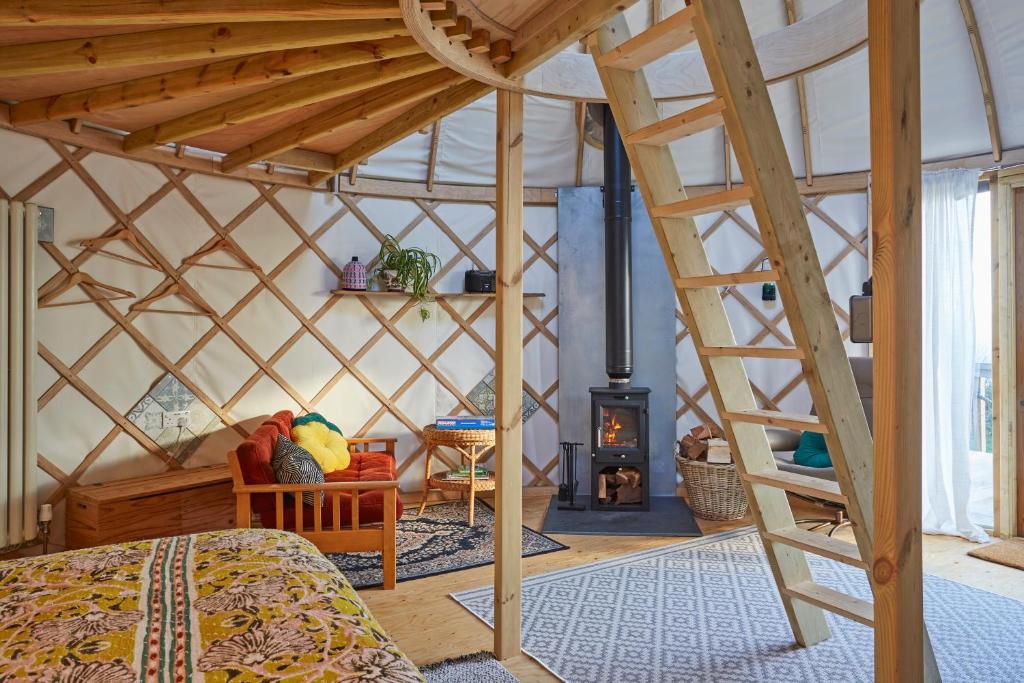The image captures a uniquely cozy bedroom with a rustic charm, framed predominantly in wood. The main focal point is a bed adorned with a yellow floral comforter, surrounded by wooden beams and a crisscross wood design against the wall, and sheltered by a darker wooden roof overhead. A ladder positioned in the middle of the room ascends to an upper loft area. Adjacent to the bed is a small couch with a vibrant red velvet cushion, decorated with a collection of throw pillows in yellow, green, and a black-and-white stripe pattern. 

In the corner, a vintage black wood-burning stove sits with its pipe extending upward into the chimney. The floor showcases an area rug at the base of the ladder, and in front of the bed, another rug adds to the room's warmth. A nearby wooden shelf, adorned with greenery and various knickknacks, adds a homey touch, while a wooden chest provides additional storage. 

A straw-like rattan coffee table stands beside the couch, and a small stool with a book rests nearby. The room is decorated with white curtains that hang in the distance, partially obscuring what appears to be a doorway that might lead out to a balcony. Hangers and a basket with various items are also visible, enhancing the rustic and eclectic ambiance of the space.